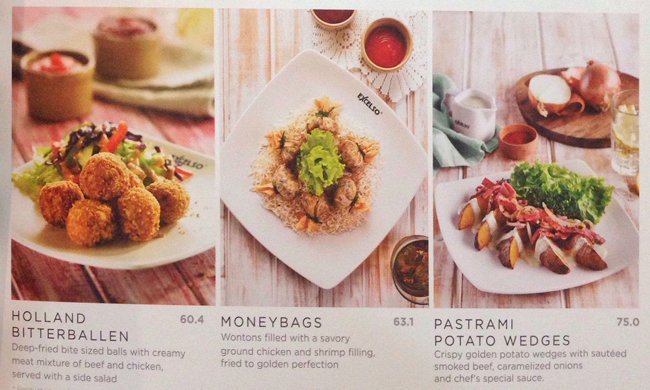This is a color photograph in landscape orientation, portraying a page from what appears to be a high-end restaurant menu. The page features three side-by-side images of different food dishes, each accompanied by detailed descriptions beneath them, set against a light gray background.

On the left, there's a white plate holding small, round, deep-fried balls called "Holland Bitterballen." These bite-sized snacks have a creamy meat mixture of beef and chicken and are served with a side dish. The description includes a price of $60.40. 

In the center, another white plate is shown from above, holding "Moneybags." These are wontons filled with savory ground chicken and shrimp, fried to a golden perfection, and served with dipping sauces. The price mentioned is $63.10.

The image on the right features a white plate with crispy golden potato wedges, a green salad, and sautéed smoked beef with caramelized onions, labeled as "Pastrami Potato Wedges." The price for this dish is $75.00. Behind this plate is a wooden cutting board with a halved onion and other food items, enhancing the rustic appeal.

The menu design utilizes earth tones of green, red, and brown, giving it a laid-back yet refined aesthetic in both the food presentation and the accompanying graphic design typography.